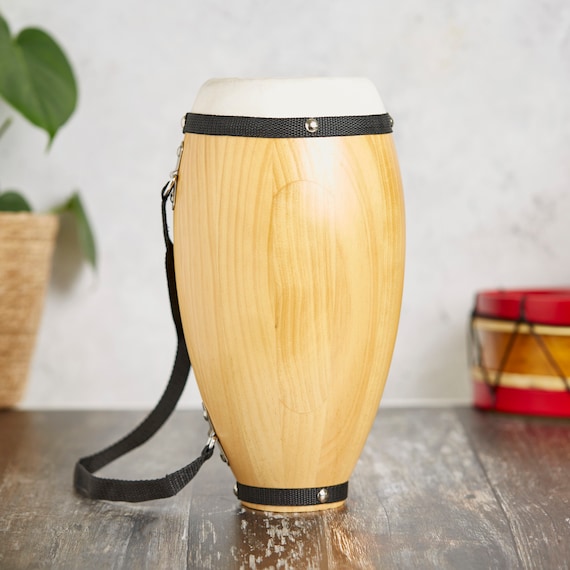The image showcases a bongo drum prominently positioned at its center. The bongo features a highly polished wooden base of a light bamboo color, transitioning to a taut, white drumhead. Encircling the junction of the drumhead and base is a black, corded strap with decorative elements, highlighting its craftsmanship. This strap extends down the left side, connecting to another strap designed for portability, allowing the drum to be carried over the shoulder or around the neck. The bongo is placed on a dark brown, hardwood floor that, despite its smooth polish, displays signs of wear with scattered scuffs and rough patches, hinting at years of use. In the background, a white wall provides a neutral backdrop. To the left, a portion of a plant in a wicker pot introduces a touch of greenery, while on the right, a red drum with a wooden base can be seen resting against the wall. The meticulous arrangement of these elements suggests the image may have been staged, potentially for a website.